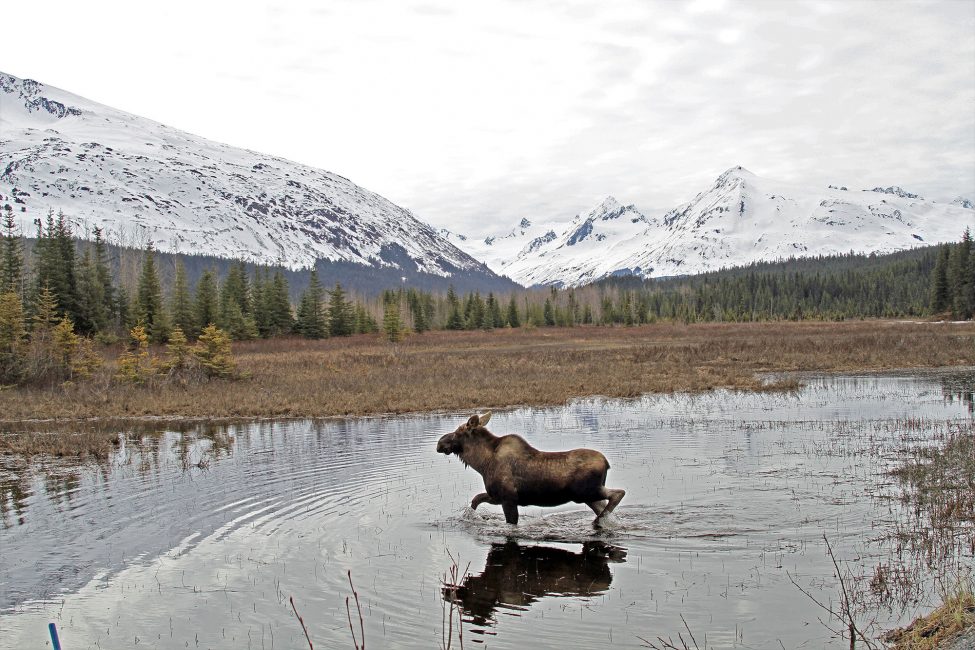In this detailed landscape photograph, a brown, antlerless moose is captured wading through a shallow creek with gray, calm water. Positioned toward the bottom center of the image, the moose is moving from right to left, with its two front legs lifted and splashing water, creating a sense of motion. Its long snout and the characteristic hump over its shoulder are clearly visible. Below the moose, its reflection shimmers on the water's surface.

Beyond the creek, the landscape transitions into a large field of brown, flat grass. Further back, there is a ring of conical-shaped trees, a mix of green evergreens and some brown, stretching from the left to the right of the image. These trees form a natural boundary before giving way to a stunning mountain range. The mountains, blanketed in snow, feature a gradient from soft, rounded inclines on the left to more rugged, craggy peaks on the right, separated by a gentle valley in the middle.

The sky above is primarily white and cloudy, with a glare noticeable from the middle of the top extending to the left side of the image. The overall scene captures the serene beauty of the wilderness, with the moose being the central focus amid the expansive natural backdrop.